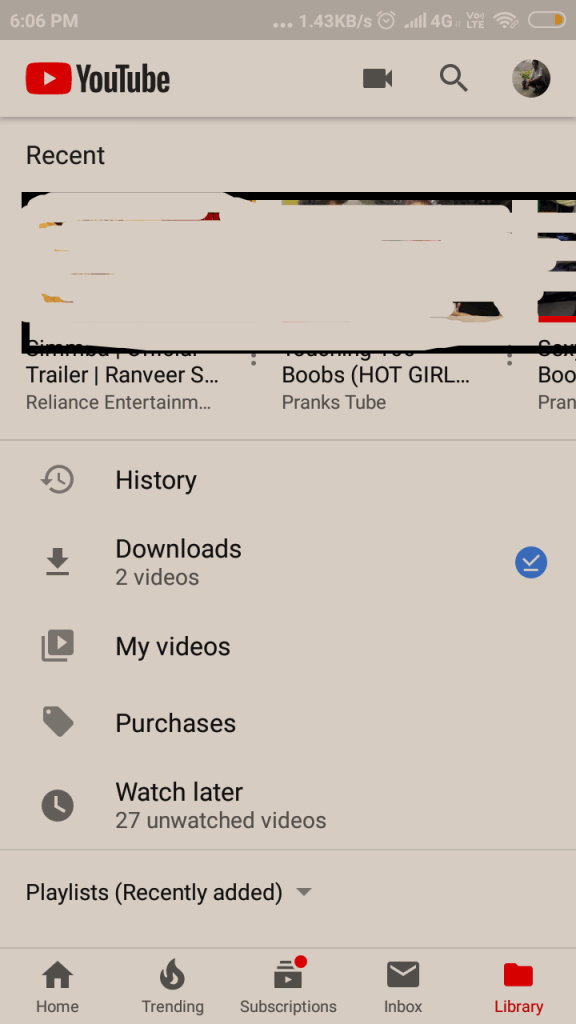This screenshot captures the main screen of the YouTube mobile app. At the top, the iconic YouTube logo is prominently displayed with its signature red rectangle and white play button. On the right side of the logo, three icons are visible: a video camera, a magnifying glass, and a circular profile picture featuring a silhouette of a person facing left.

Below this toolbar, a "Recent" section showcases partially visible thumbnails of recently watched videos. The first visible video is labeled "Trailer" and is uploaded by Opera Lines Entertainment. The next video, from PranksTube, is partially obscured, and another thumbnail is cut off on the right side of the screen.

Further down, a menu with five options is visible. It includes:
1. History
2. Downloads - indicating two videos have been downloaded
3. My Videos
4. Purchases
5. Watch Later - currently listing 27 videos.

The detailed elements in this screenshot provide a comprehensive view of the user's navigation options and recently viewed content on YouTube.